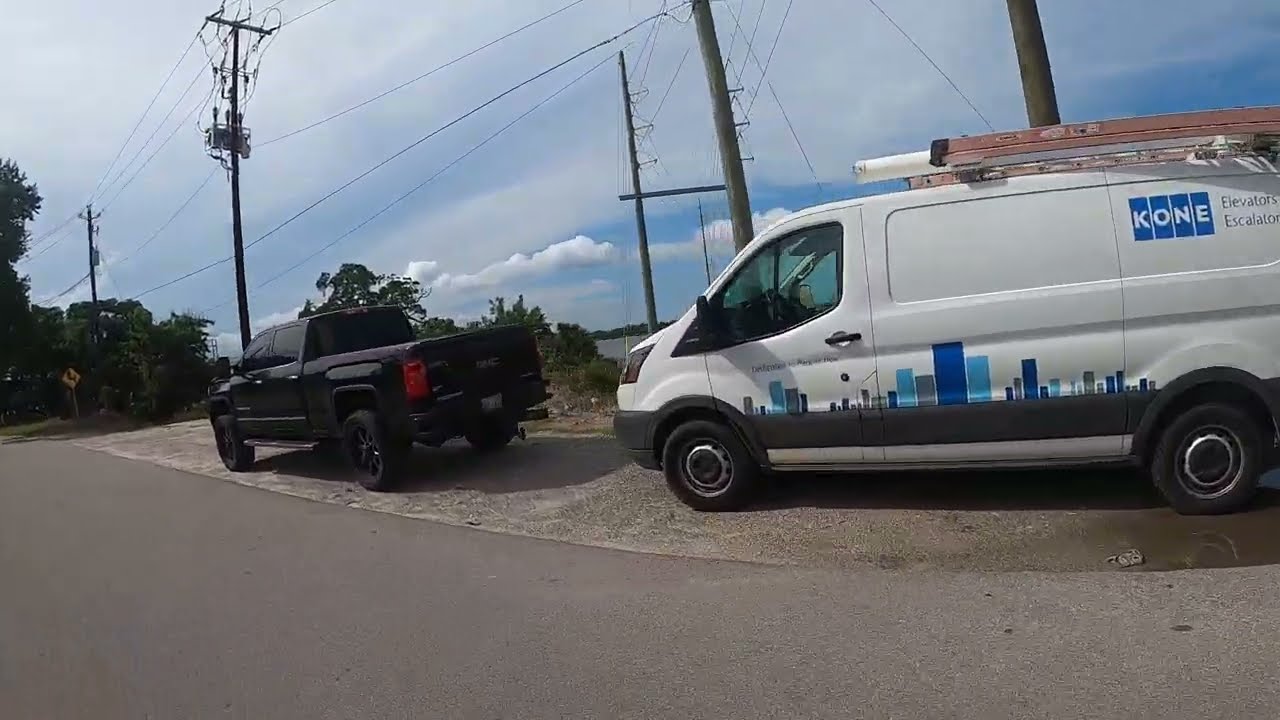In this photograph, a white van and a black pickup truck are parked side by side on the edge of a gray paved road, both facing to the left. The black pickup truck features red taillights and has black wheels, while the van, with silver-rimmed black wheels, prominently displays the company name "KONE" in white letters on four blue rectangular panels on the right side. Below this, the words "Elevators and Escalators" are written in black. The van is adorned with an illustration of a blue city skyline along its lower sides, and a brown ladder is secured to its roof. The scene is set against a backdrop of numerous wooden telephone poles with power lines stretching across the image. To the left of the frame, green trees and a yellow diamond road sign—whose message is unreadable—are visible. Overhead, the sky is light blue, filled with thin, diffuse white clouds.